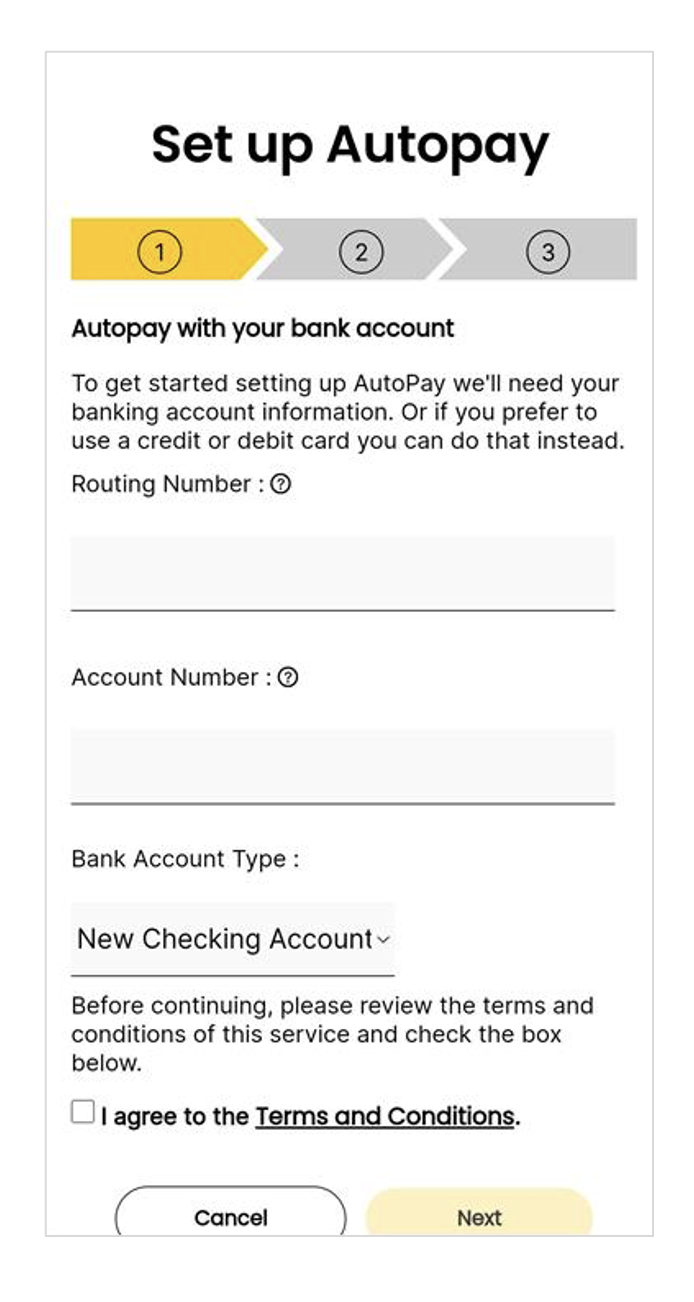The image is a screenshot from a smartphone with a vertical orientation, featuring a user interface for setting up auto pay on a white background. At the top of the page, bold black text prominently displays the title "Set Up Auto Pay." Directly beneath this title, there is a visually distinct banner composed of three numbered sections, each bearing an arrow pointing to the right, outlining the sequential steps required to set up the auto pay feature. 

The first section is marked with a yellow color and numbered "1," the second section is numbered "2," and the third section is numbered "3." This step-by-step banner visually guides the user through the process. 

Below this banner, the text "Auto Pay with Your Bank Account" introduces the main content area. There is an instructional message indicating the need for banking account information to set up auto pay, with an option to use a credit card or debit card if preferred. 

The interface includes fields for entering banking details. Firstly, "Routing Number" is labeled, accompanied by a small question mark within a circle that likely provides additional information. Adjacent is an empty text box designated for the routing number input. Below this, "Account Number" is similarly labeled, followed by another question mark within a circle for detailed guidance and an adjoining text box for the account number entry.

Further down, the text "Bank Account Type" appears above a rectangular drop-down menu, currently displaying "New Checking Account," with a right-pointing arrow for selecting different account types.

Before progressing, users are prompted to review the service's terms and conditions, which are specified in an italicized and underlined text link. An empty checkbox precedes the statement "I agree to the terms and conditions," signaling user agreement is required to proceed.

Finally, at the bottom of the screen, two buttons are present: a white "Cancel" button on the left, and a yellow "Next" button on the right, enabling users to either exit the setup or continue to the next step.